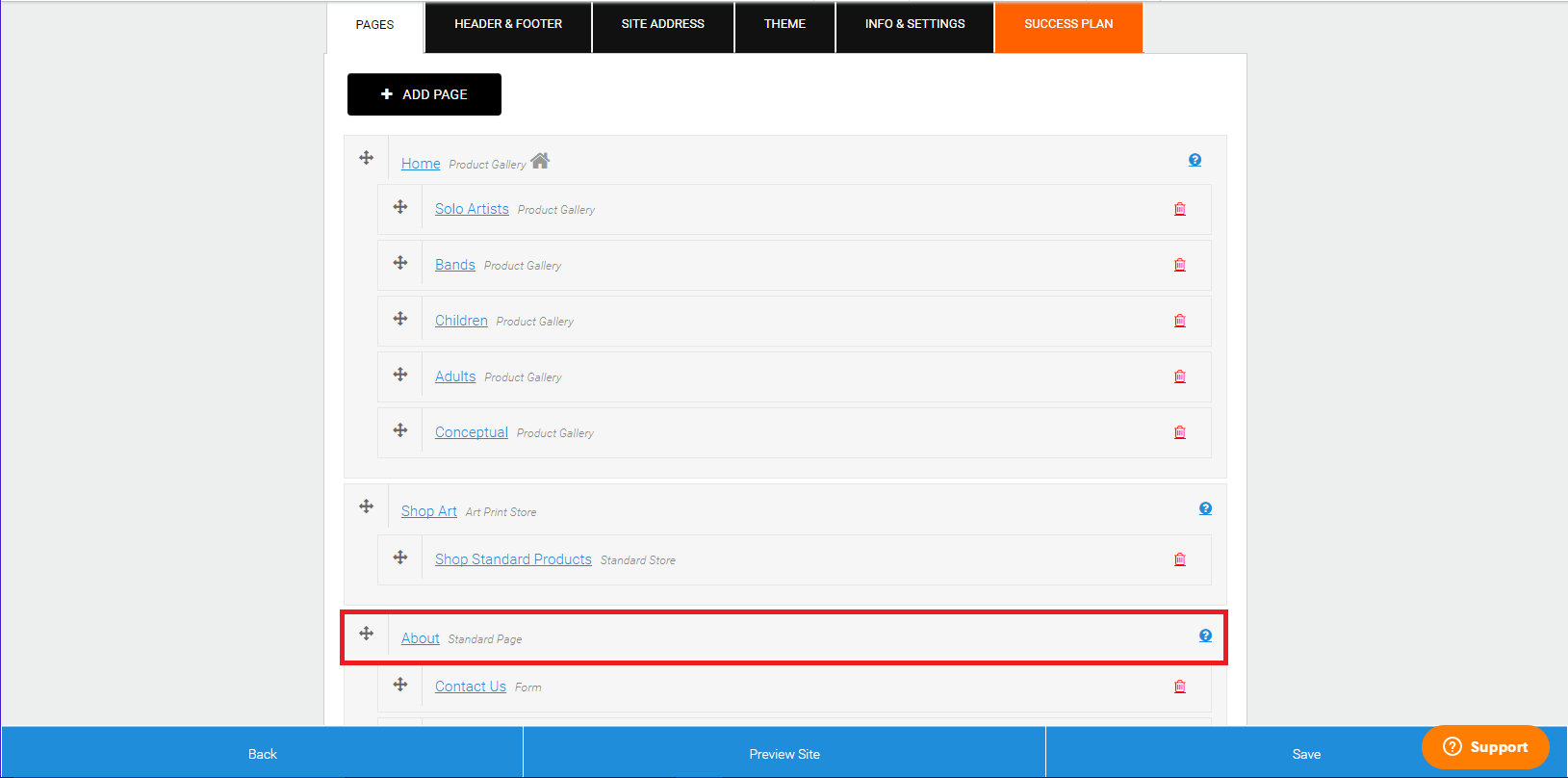Caption: "The website interface displays a navigation bar at the top with several headings: 'Pages', 'Header and Footer', 'Site Address', 'Theme', 'Info and Settings', and 'Success Plan'. The 'Pages' heading is white, indicating it is currently selected. The other headings are in black, except for 'Success Plan' which is orange. On the 'Pages' section, an 'Add Page' button with a black plus icon is visible at the top. Below this, a hierarchical structure lists categories such as 'Home', 'Solo Artists', 'Bands', 'Children', 'Adults', 'Conceptual', and subcategories like 'Shop Art', 'Shop Standard Products', along with 'About' and 'Contact Us'. A red rectangle highlights the 'About' section. At the bottom of the screen, a blue panel contains buttons for 'Back', 'Preview Site', and 'Save'. In the bottom right corner, there's an orange 'Support' button with rounded edges."